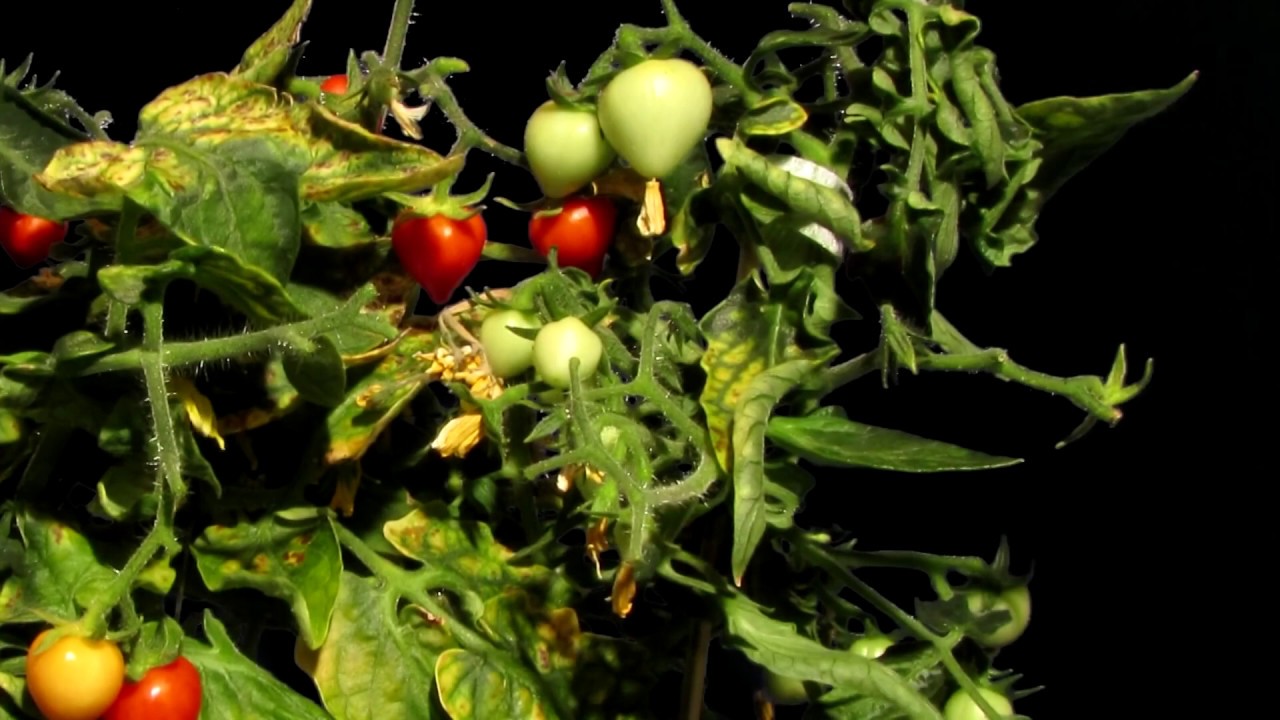The image showcases a tomato plant set against a stark black background, vividly focusing on the plant's various stages of growth. Fuzzy stems and leaves with a mix of vibrant green, yellow, and browning edges suggest parts of the plant are in distress and need pruning. Scattered symmetrically from left to right, the plant bears tomatoes in different stages of ripeness: four small green tomatoes, five ripened red tomatoes, and one yellow tomato next to a red one at the bottom left. Creeping amongst the foliage, hints of orange tomatoes can also be seen. The contrast between the tomatoes' colors and the dark backdrop makes the plant stand out prominently, capturing the viewer's attention.